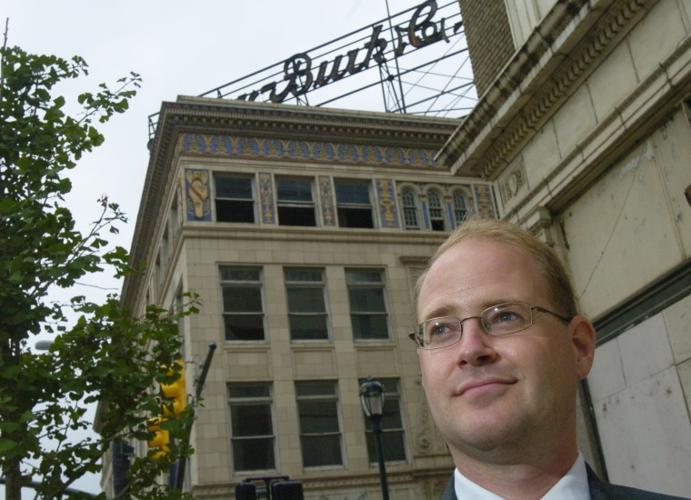This image captures a Caucasian man, likely in his late 30s to early 40s, standing outside an ornate beige stone building. The man, positioned in the bottom right corner of the frame, has thinning blonde to brown hair, wire-rimmed square glasses with a reflected light dot on each lens, and is clean-shaven. He's wearing a tuxedo or suit with a white collar visible, and he's smiling slightly as he looks to the left. Behind him, the building extends upwards for three to four stories, featuring a roof that juts out and detailed blue and gold tilework or patterns near the top, along with several open windows. At the summit of the building, a partially obscured sign displays the letters "B," "U," "R," "K," suggesting it might say "Burke." To the left side of the image, a green deciduous tree with dense foliage and a pair of yellow traffic lights add further context, indicating the man is near an intersection in front of this older, possibly historic building. Additionally, a street lamp is visible next to his right ear.